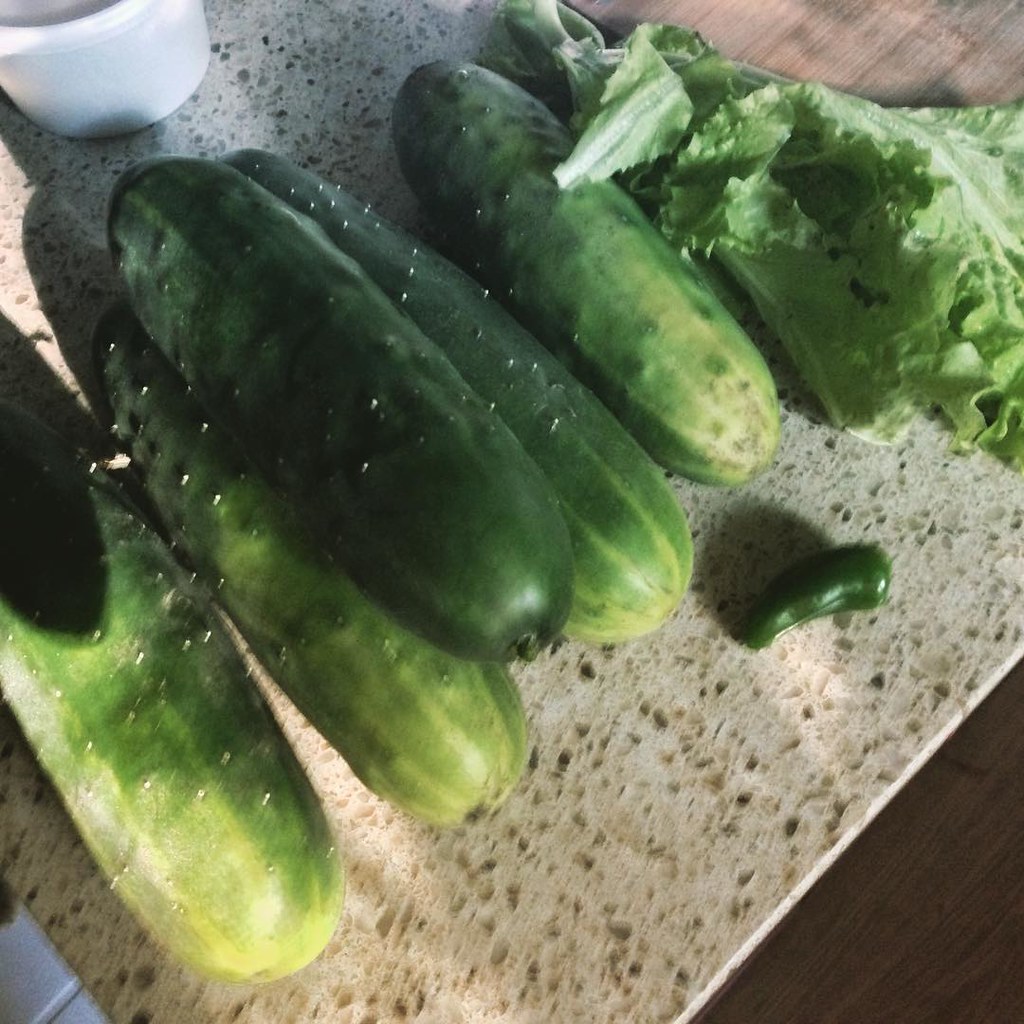This is a detailed square color photograph taken from above, showcasing an array of green vegetables on a cutting board with a speckled, flat surface consisting of gray and beige pebbles. The cutting board is positioned atop a wooden surface, visible on the upper left, upper right, and bottom right corners of the image. Central in the photo are five cucumbers, four of which lie underneath a fifth one, all arranged at a diagonal angle. The cucumbers exhibit various shades of green, with some showing darker green shading and light green spots, and one showing slight bruising. In front of the cucumbers sits a small green jalapeño pepper. Off to the right, partially resting on both the cutting board and the wooden surface below, is a piece of green lettuce, potentially iceberg. Adding to the composition, a small white souffle cup is positioned in the top left portion of the image. A natural shadow cast on the cutting board suggests the presence of natural lighting, possibly from a nearby window.